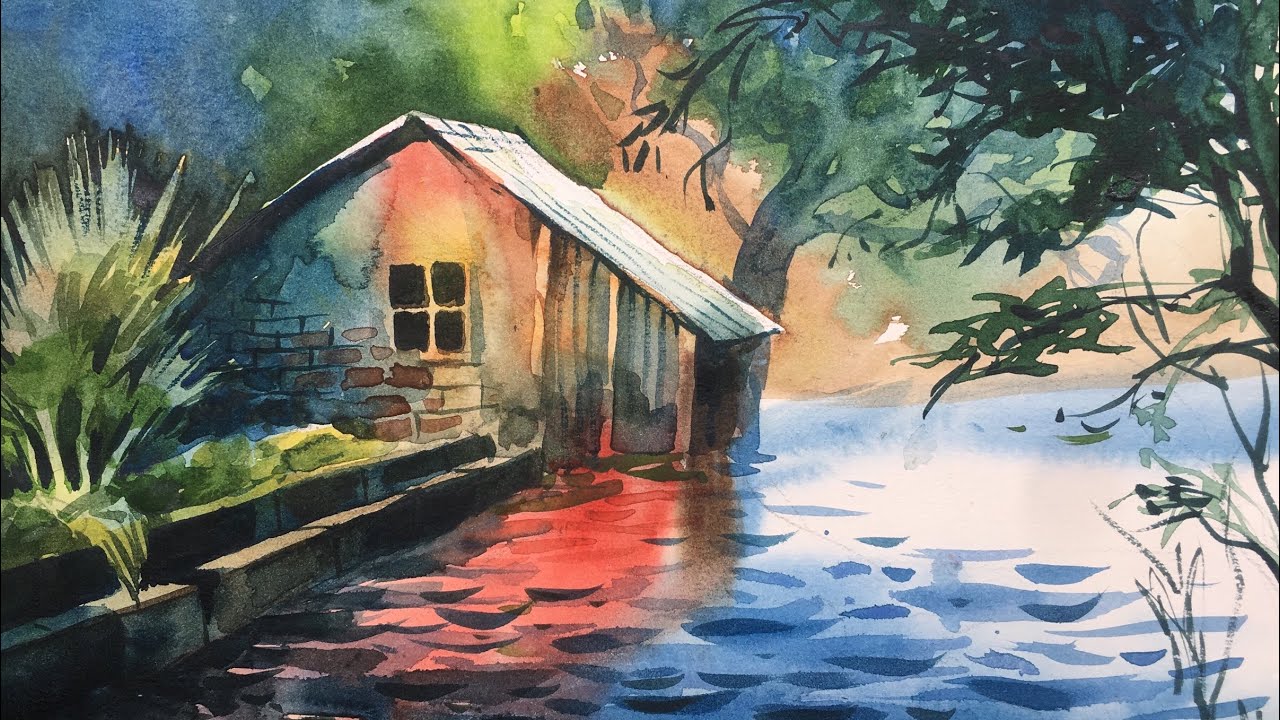This watercolor painting depicts a quaint, old brick house with wooden elements and a small single window. The house, which resembles a shed with possibly a tin roof, is set against a backdrop that suggests night, with a dark blue sky enhancing its muted tones. Attached to the right of the house is a shed area, while to the left, a very large garden bed stretches out, filled with low greenery and spiky bushes. Beyond the house, there's an abundance of trees, with a particularly large tree standing prominently beside it. The ground in front of the house is painted in blue-grey hues, which can be interpreted as either a cobblestone road or gentle waves of water. The varied palette includes greens, blues, reds, and browns, creating a harmonious blend that captures the serene atmosphere. The meticulous blending of these colors adds to the ambiguous yet captivating nature of the scene.